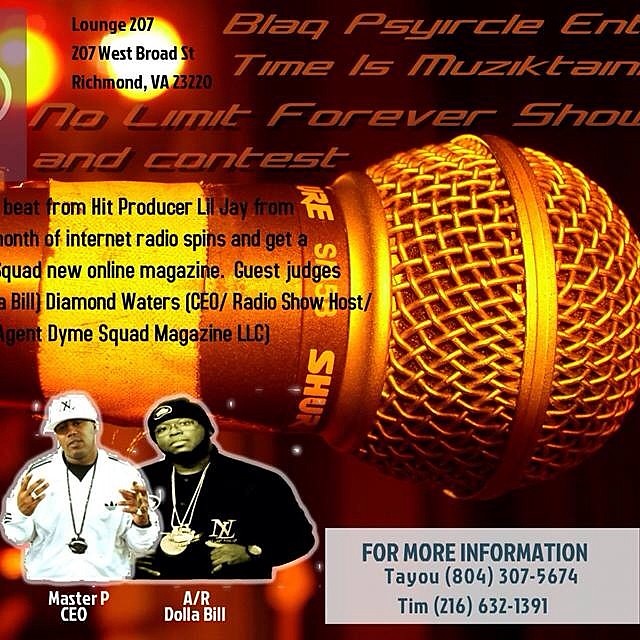Here's the revised and detailed single caption:

This promotional poster for a rap show at Lounge 207, located at 207 West Broad Street, Richmond, Virginia, 23220, features a prominent image of a horizontal microphone in a bright, yellow-gold hue. Near the top left corner, the text reads "Lounge 207, 207 West Broad Street, Richmond, Virginia, 23220." Below that, the names of performers are listed: Black, Psyche, Time Is Mute, T-A-I-N, Teal, No Limit Forever Show, and Contest. The poster also mentions hit producer Lil J, and highlights involvement from new online magazine guest judges, including Bill J. Diamondwater, CEO of Hunt Dying Squad Magazine, LLCJ. 

Beneath the microphone image, there are photographs of two black men. The first, wearing a white sweater, necklace, and baseball cap, is identified as Master P, CEO. Next to him, a man in a black jersey, black stocking cap, and wearing medals is labeled AR Dollar Bill. In the bottom right corner, there is additional contact information in gray and blue: for inquiries, call 804-307-5674 or Tim at 216-632-1391.